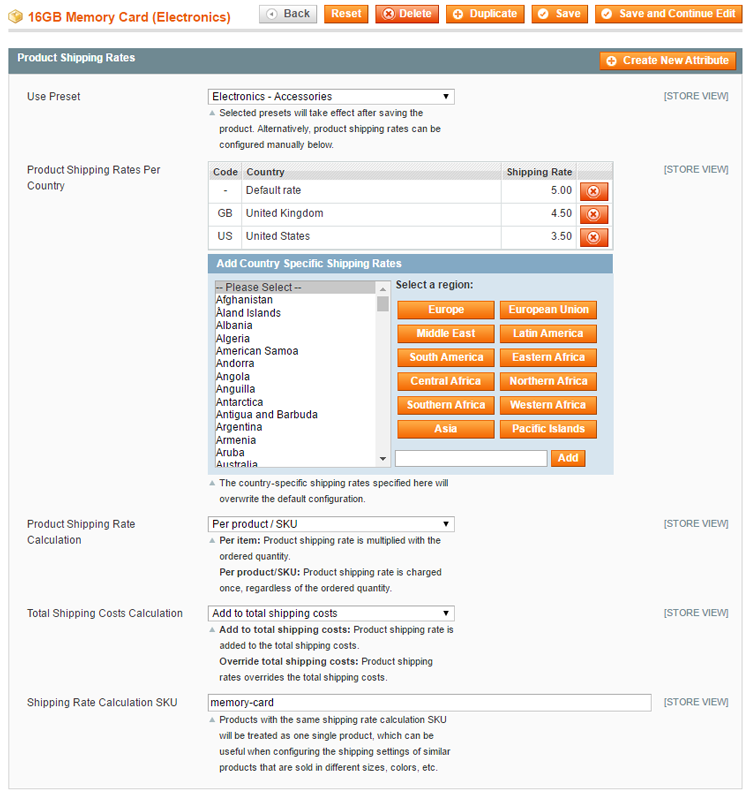The image displays the interface of an online shopping site where a user is browsing for a 16GB memory card, prominently featured in the top left-hand corner. The interface includes a series of clickable icons on the top row, styled as orange rectangles, labeled 'Save and Continue,' 'Edit,' 'Save,' 'Duplicate,' 'Delete,' and 'Reset.' Additionally, a silver 'Back' button is located to the left.

In the product shipping section, the user has selected 'Electronics' and 'Accessories.' There is also an option to create new attributes. Below this section, there is a dropdown menu where users can choose the country for setting shipping rates. Currently, the United Kingdom and the United States are selected. The shipping rate for the United Kingdom is set at $4.00 or $4.50, whereas for the United States, it is set at $3.50.